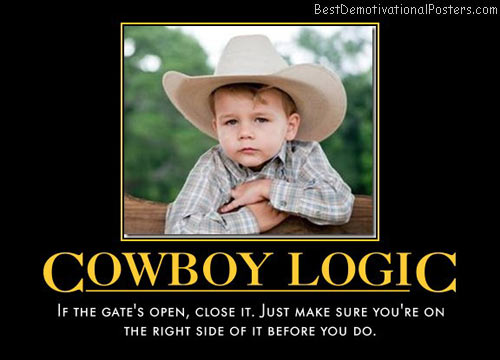The meme features a demotivational poster with a central photo of a young boy, approximately five or six years old, wearing a large white cowboy hat and a gray, patterned, collared, long-sleeve shirt. The boy, who is light-skinned, is leaning and slumped over a wooden fence beam, with blurred trees in the background set against a hazy sky. He looks calm and is staring straight ahead. Below the photo, in large yellow all-caps letters, it says "COWBOY LOGIC," and underneath that, in smaller white letters, it reads, "IF THE GATE'S OPEN, CLOSE IT. JUST MAKE SURE YOU'RE ON THE RIGHT SIDE OF IT BEFORE YOU DO." The entire image is framed by a plain black background, and in the upper right corner in small white letters, it reads, "BEST DEMOTIVATIONAL POSTERS DOT COM."